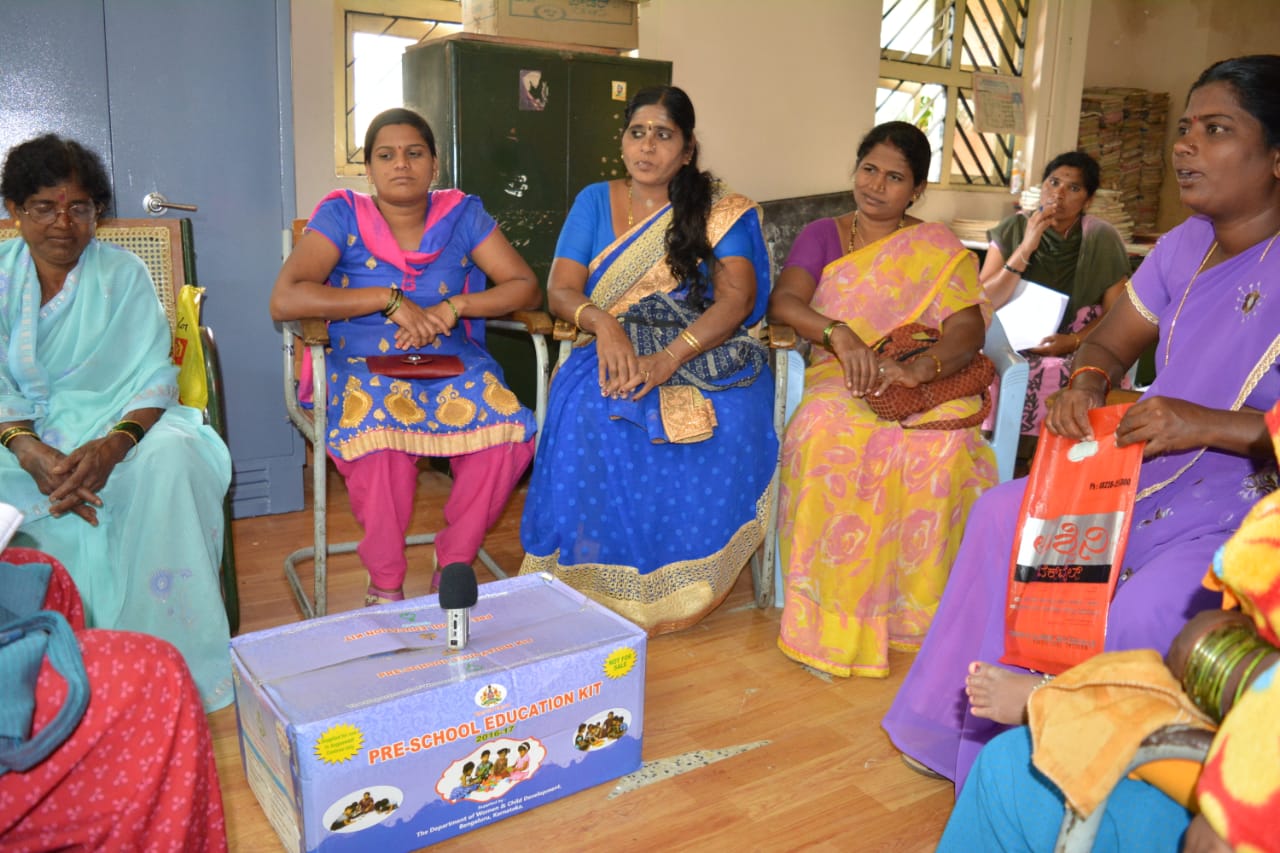This photo captures a group of eight Indian women, all dressed in vibrant traditional attire, sitting in a semi-circle inside a room with blue and white walls and a cabinet in the background. Most of the women are wearing numerous bracelets, and several hold purses or wallets on their laps. In the center of the group is a box labeled "Preschool Education Kit," with a microphone placed on top, suggesting they might be recording or broadcasting a session. The women, adorned in dresses of various bright colors such as purple, yellow, pink, light purple, and dark blue with gold accents, are engaged in what appears to be a discussion or interview. One woman is holding a red bag with writing on it, possibly just returning from a store, and is speaking. Another woman towards the back, who might be smoking or touching her lips, looks directly at the camera. The composition of the scene suggests a thoughtful and vibrant communal interaction.